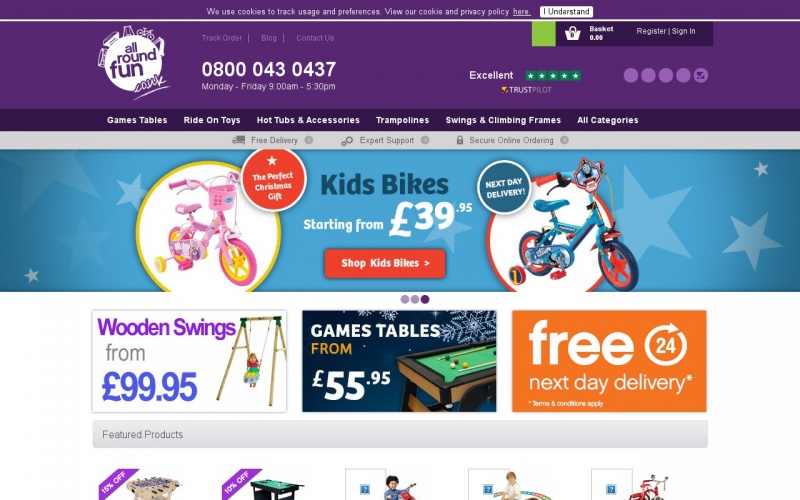The webpage from "All Around Fun"—an online retailer specializing in outdoor and recreational products for kids and families—features a well-organized and engaging design. At the top, there is a banner that notifies users about the website's use of cookies for tracking usage and preferences, with a link to the cookie and privacy policy, accompanied by a consent button labeled "I Understand" on the right side. In the top-right corner, there are links for "Register" and "Sign In" along with a basket icon. Notably, the registration should be restricted to adults.

The header includes the “All Around Fun” logo and a contact number, 0800-043-0437, with service hours listed as Monday to Friday, 9 a.m. to 5:30 p.m. Additional links for tracking orders, accessing the blog, and contacting customer service are visible. TrustPilot ratings with star icons and an "Excellent" rating are also highlighted, reinforcing the site's credibility. Main navigation covers product categories including "Games Tables," "Ride-On Toys," "Hot Tubs and Accessories," "Trampolines," "Swings and Climbing Frames," and a comprehensive "All Categories" section.

The main content area prominently features a promotional banner for kids' bikes starting at $39.95. This banner positions the bikes as the perfect Christmas gift and highlights the option for next-day delivery. The colorful images of pink and blue kids' bikes and a "Shop Kids' Bikes" call-to-action button command attention.

Secondary promotional banners are positioned below, with the left banner advertising wooden swings starting from $99.95, featuring an image of a wooden swing set. The center banner promotes games tables starting at $55.95, including a picture of a pool table. The right banner emphasizes free next-day delivery within 24 hours, with terms and conditions applying, indicated by an asterisk.

Further down, the "Featured Products" section displays various toys and equipment, though the images are somewhat indistinct. Among them, a foosball table and a hockey table can be discerned. The footer includes links and icons for social media and additional contact details.

The website uses a vibrant and kid-friendly color scheme with purple and blue hues accented by white text. Bright colors and playful fonts underscore the focus on children’s products and family fun activities, making the site visually appealing and inviting for its target audience.